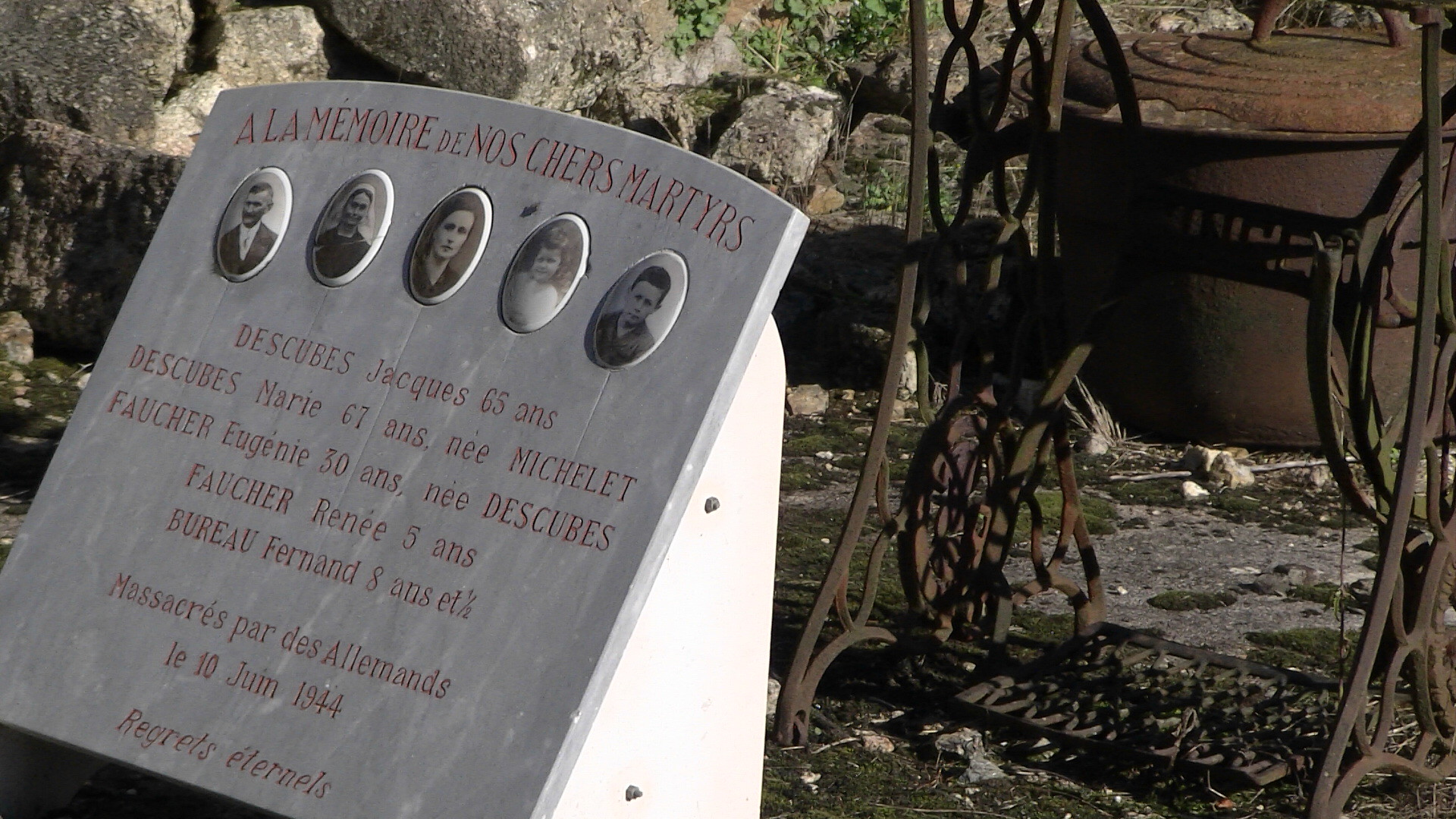This photograph, taken outdoors during what looks like the late afternoon near sunset, captures a somber scene set in a historical or memorial site. The main focus is a rectangular, gray marble plaque with red lettering, positioned on the left-hand side of the image. The plaque, which is quite thin and has a slightly rounded top, bears a prominent title in red that reads "À la mémoire de nos chers martyrs" (In memory of our dear martyrs). Below this, the plaque features elongated oval portraits of five individuals—a 65-year-old man named Jacques, a 67-year-old woman named Marie, a woman in her 30s named Eugénie, a 5-year-old girl named Renée, and an 8-year-old boy named Fernand. The French inscription at the bottom indicates that they were massacred by the Germans (par des Allemands) on June 10, 1944, followed by the phrase "regrets éternels" (eternal regrets).

Set against a backdrop of large stone and rock formations, the plaque sits next to a rusted old tool or carriage on the right side of the image. The ground around these objects is a mixture of grass and stones, contributing to the historical ambiance. Additionally, an old stone pot on a stand is visible on the right-hand side, reinforcing the site's aged and rustic atmosphere. The image overall feels very poignant, capturing the essence of remembrance and loss.